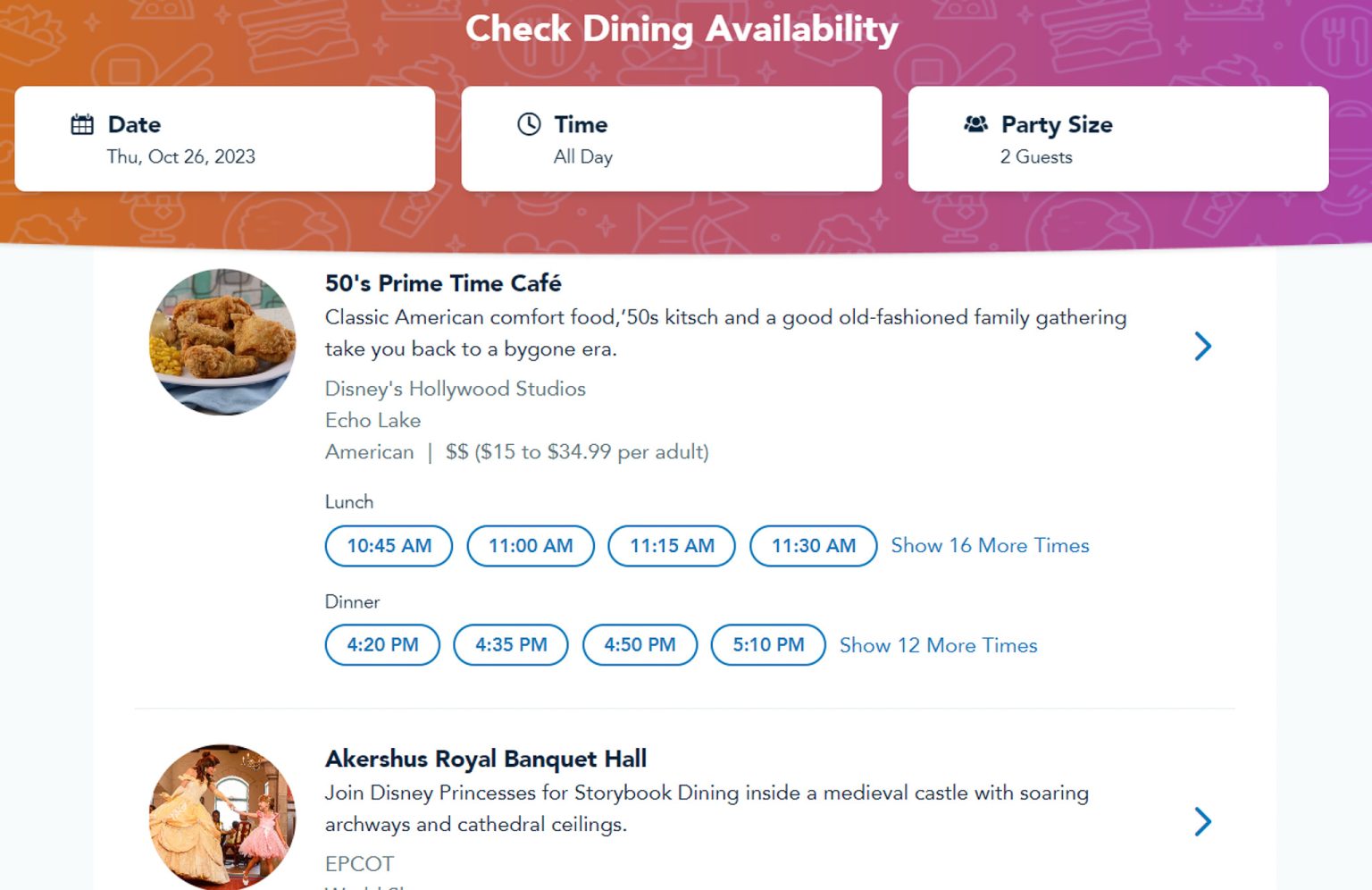In this image, there are details about dining options at Disney's Hollywood Studios. The primary focus is on dining availability for a party of two guests on Thursday, October 26th, 2023. One of the featured restaurants is the 50's Prime Time Café, known for serving classic American comfort food in a 1950s-themed setting filled with kitsch and nostalgia, resembling a good old-fashioned family gathering. The price range for this dining experience is between $15 to $34.99 per adult.

Additionally, there is also information about Acacia's Royal Banquet Hall, where guests can enjoy storybook dining with Disney princesses. This restaurant is situated inside a grand medieval castle adorned with soaring archways and cathedral ceilings. Both dining venues offer unique experiences, with 50's Prime Time Café evoking a bygone era of American culture, and Acacia's Royal Banquet Hall providing an enchanting atmosphere.